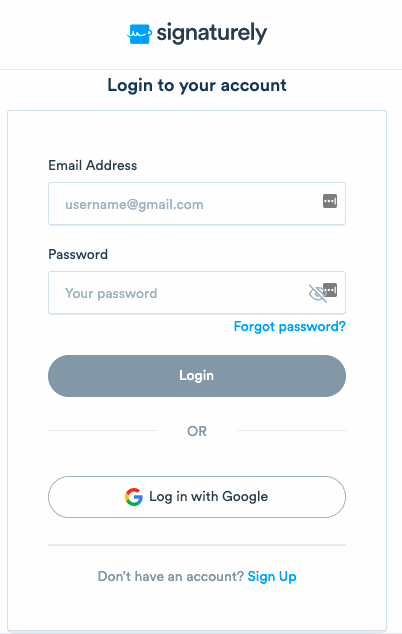The login page for an account on the Signaturely website features a clean white background with a blue square logo centered at the top. The logo consists of a stylized squiggly line resembling the letter "M" with a heart at the end on the right. Next to the logo, the brand name "Signaturely" is displayed in bold, lowercase black lettering. A gray horizontal border extends across the screen beneath the logo and text. 

Following the border, the title "Log in to your account" is presented, with a slight space below it. Another gray border frames the login section of the page, running horizontally from left to right and vertically along the left side and bottom. 

Within this section, the text "Email address" is prominently bolded in black, followed by a rectangular input field that suggests entering an email address, displayed in gray as "username@gmail.com." Adjacent to the input field, on the left, is a small square icon with three ellipses and a white line down the right side.

Next, the text "Password" appears in black above another rectangular input field labeled "Your password." To the left of this field is a similar small square icon; to the right, there is an eyeball icon with a diagonal line indicating "Show/Hide Password."

Beneath the password field, the link "Forgot password?" is displayed in blue on the right side. Below this, a large gray button with white text reads "Log in." 

Centered underneath the button is the word "Or," flanked by gray horizontal lines on either side. Following this, a white button with the Google "G" logo is captioned "Log in with Google."

At the very bottom, the text "Don't have an account?" appears in gray, followed by a blue "Sign up" link, encouraging new users to create an account.